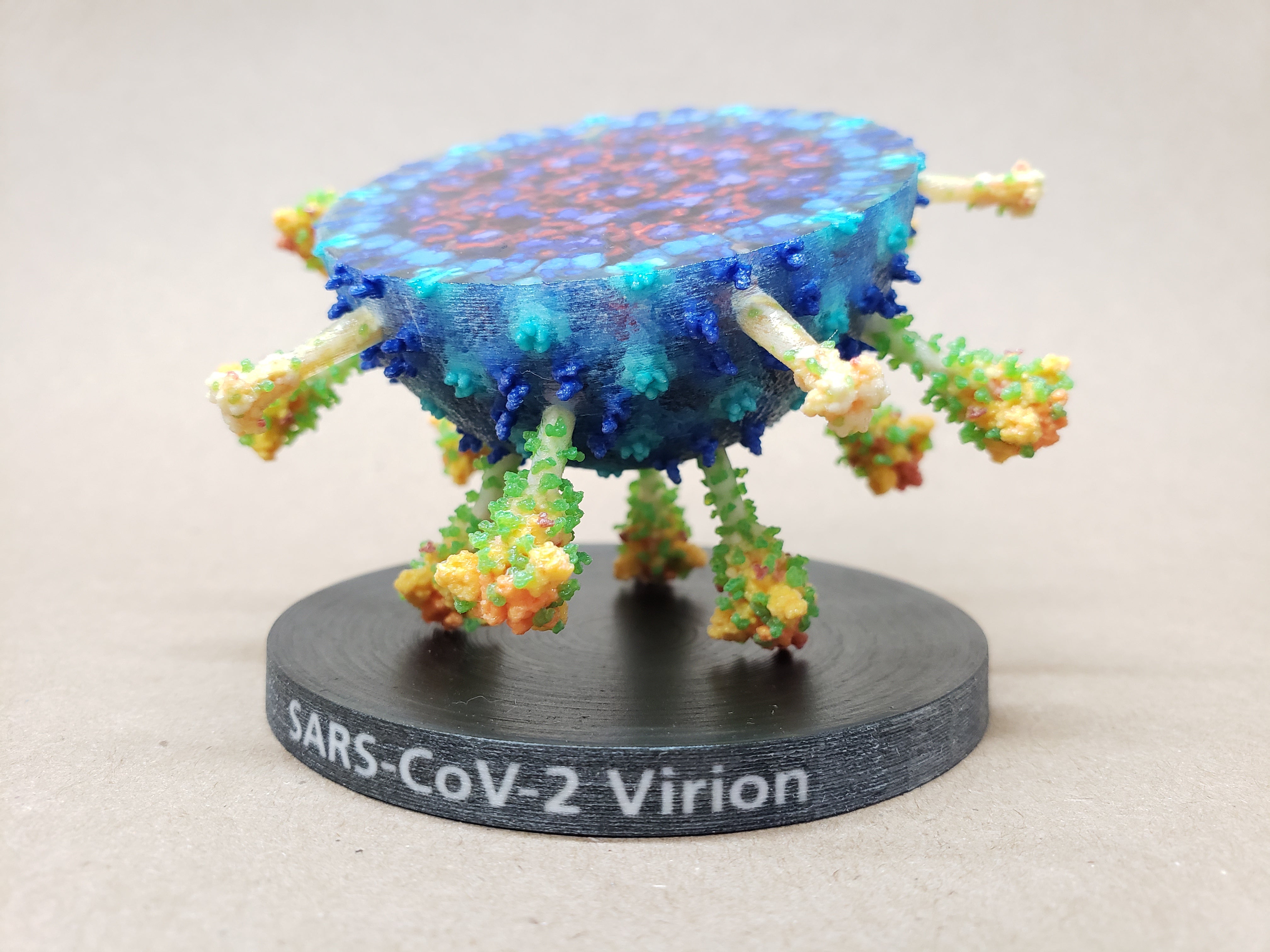The image depicts a 3D printed model of the SARS-CoV-2 virus, distinctly showcasing its structure in a detailed and visually striking manner. The model, which is cut in half to reveal the interior, is prominently mounted on a black pedestal labeled "SARS-CoV-2 Virion." The virus is shaped like a half sphere, with the outer part rendered in various shades of blue, accentuated by spikes that exhibit a mix of yellow, green, beige, and orange colors. The interior is rich with colors such as red, purple, and light blue, highlighting the complex inner components. The model distinctly exhibits the texture typical of 3D printing, apparent through the layered plastic build-up both on the virus itself and the pedestal. The background is plain, either beige or gray, ensuring the focus remains solely on the intricate details of the virus model and its academic presentation. The sculpture stands out against the minimalistic backdrop, clearly showcasing the virus that causes COVID-19.